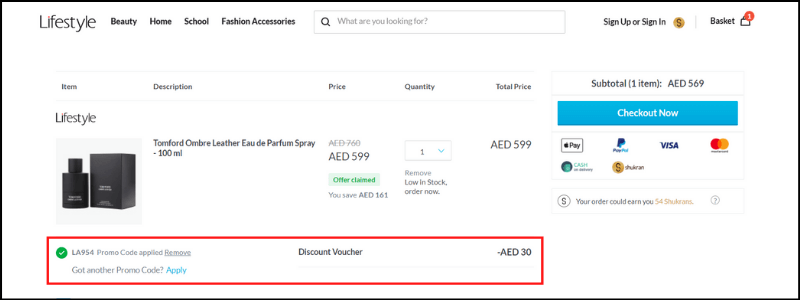This detailed and comprehensive caption describes the various elements visible in an online store interface:

---

The image depicts the interface of an online store set against a white background. At the top, there's a header with various tabs. Beginning from the left, the tabs are labeled: "Lifestyle," "Beauty," "Home," "School," "Fashion Accessories," followed by a search bar with the placeholder text, "What are you looking for?"

On the top right, there's an option to "Sign Up" or "Sign In," adjacent to an orange icon of a shopping basket. The basket shows a small red indicator with the number '1,' indicating one item is currently in the basket.

Moving below, on the right side of the page, it displays a summary section. Here, it states "Subtotal," indicating one item priced at AED 599. A prominent blue "Check Out" button is visible near this section. Below the button, there are icons representing various payment methods: Apple Pay, PayPal, Visa, Mastercard, Cash on Delivery, and Shukran. Additionally, a note "Your offer could earn you 54 Shukrans" is mentioned.

On the left side, there is a detailed column layout under headings: Item, Description, Price, Quantity, and Total Price. The column lists one item categorized under "Lifestyle." It includes a small image of the product, which is a black box and bottle. The description reads "Tom Ford Ombre Leather Eau de Parfum Spray, 100ml." The initial price is AED 760, but it is crossed out and displayed as AED 599, showcasing a discount with the text "Offer Claimed" in green and noting "You saved AED 161."

The quantity is listed as one (with a note indicating low stock and prompting to "Order Now"), and the total price confirms AED 599. Towards the bottom, it mentions a "Discount Voucher" reducing the price by AED 30, verified with a green tick. There's also an option to "Get another promo code" and an "Apply" button outlined in red to use the promo code.

---

This caption thoroughly explains the layout and content of the illustrated online store page.